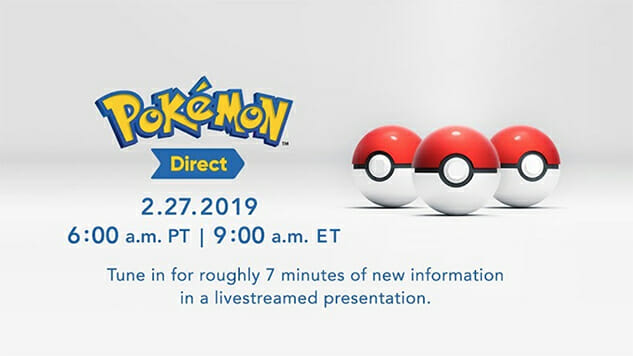This image promotes an event associated with Pokémon, specifically the Pokémon Direct presentation. The background features a gradient transitioning from a very light lilac at the top to white at the bottom. Towards the upper left, the iconic Pokémon logo is prominently displayed in its recognizable yellow font outlined in blue. Below the logo, a blue rectangular bar with the word "Direct" within it is clearly visible.

To the right of the logo and bar, there are three vivid red and white Poké Balls aligned with the central one at the front and two slightly behind. The text on the image reads: "2-27-2019, 6am PT, 9am ET. Tune in for roughly 7 minutes of new information in a live-streamed presentation." The Poké Balls and Pokémon logo serve as focal points, making the announcement visually engaging, while the clear and concise text provides essential event details.